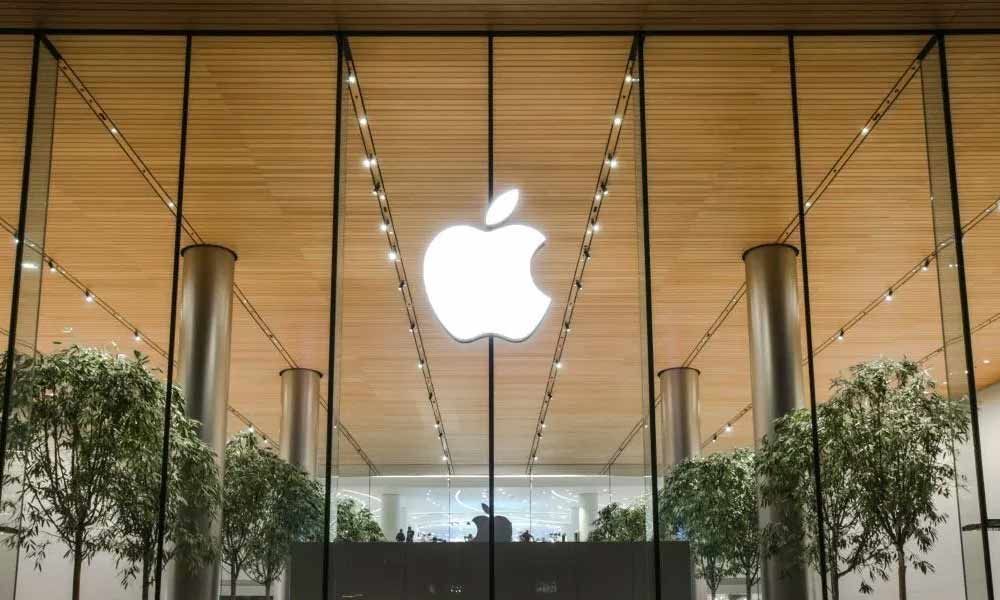This photograph captures the sleek interior of what appears to be an Apple office facility or retail store. The focal point is a spacious lobby or entryway, distinguished by a large glass wall. An illuminated Apple logo, with its iconic bite taken out, glows white atop this glass structure, symbolizing the brand's presence. The environment exudes a modern and sophisticated vibe through its golden tan wooden ceiling, which features track lighting running lengthwise to enhance the ambiance. Four substantial silver pillars support the ceiling, adding to the architectural magnificence. Scattered across the lobby are approximately six trees, possibly live or artificial, bringing a touch of nature indoors and accentuating the minimalist aesthetic Apple is known for.